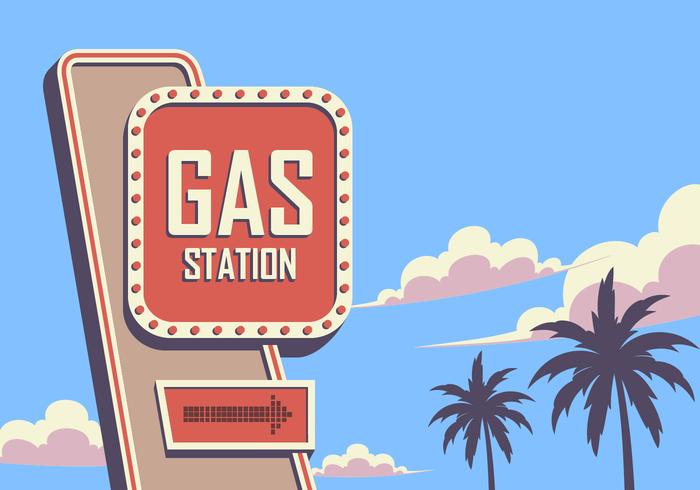The image showcases a highly stylized, modern illustration of a gas station sign set against a clear, vibrant blue sky. The sky features a few clouds that are a mix of white and a peachy pink mauve, with flat bottoms giving them a child-like, yet artistic appearance. Prominently located on the left side of the image, the gas station sign is mounted on a mauve-ish brown vertical structure, edged in red. The sign itself has white letters on a red background, surrounded by a white frame adorned with small red dots or lights. Below the main sign is another block with a black arrow, composed of dots, pointing to the right to indicate the direction of the gas station. To the right of the sign, there are two grey palm trees, adding a touch of natural elements to the otherwise sky-dominated scene. The overall design is minimalistic and has a strong, modern aesthetic, combining practical signage with artistic flair.